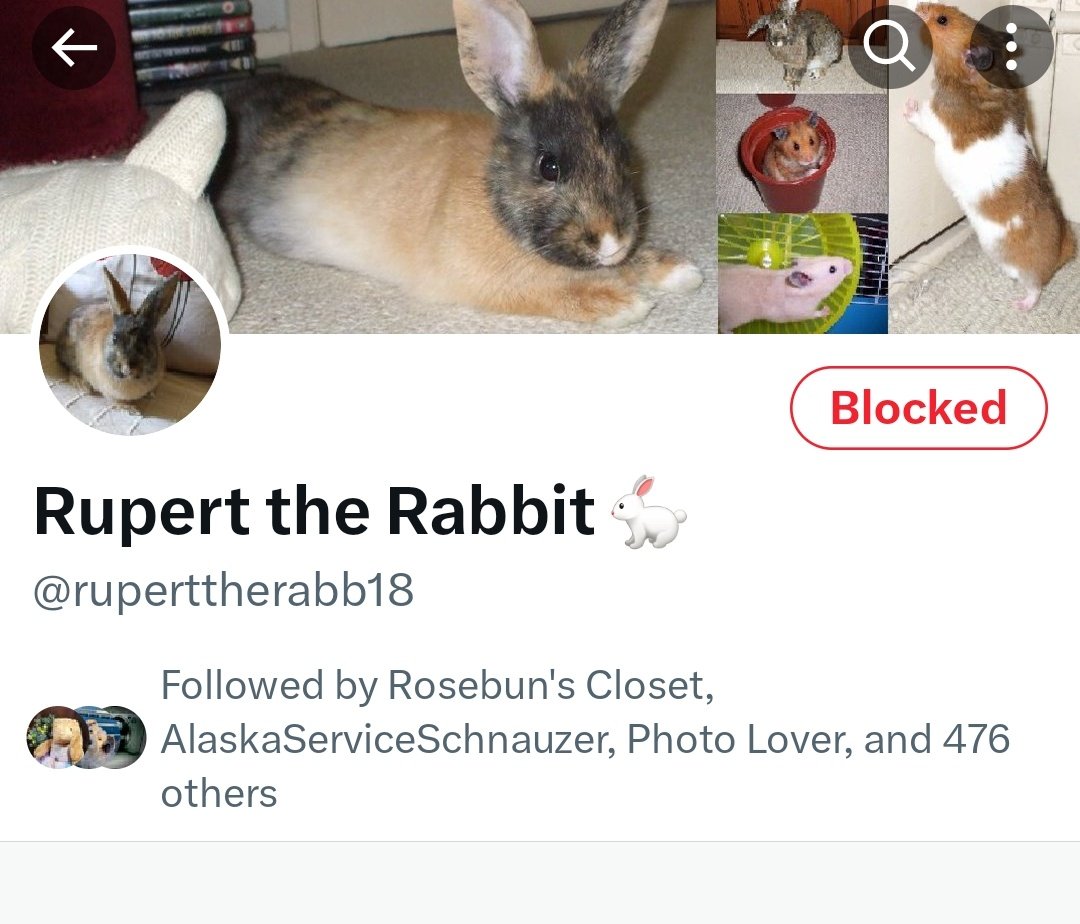In this image, we are looking at a screenshot of a social media site. At the top, there is a collection of multiple photos featuring various animals. The largest picture, placed on the left, showcases a tricolored bunny in shades of black, gold, and cream. A smaller, round picture of the same bunny, facing forward, is positioned to the lower left of the larger image. The large picture shows the bunny lying on a carpet with a stack of CDs behind it.

To the right of the large bunny photo, there are three smaller colored photos arranged vertically. The first small image is of another rabbit. Below that, the second photo captures a brown hamster sitting inside a bucket. The third photo features a cream-colored hamster running inside a yellow hamster wheel.

Further to the right, there is an image of a brown and white guinea pig standing upright, leaning against a kitchen cabinet. 

At the bottom right corner, set against a solid white background, is the word "Blocked" written in red text, displayed as a button.

Below the images, to the lower left, is the text "Rupert the Rabbit" followed by the social media handle "@RupertTheRabbit18" written in large black font.